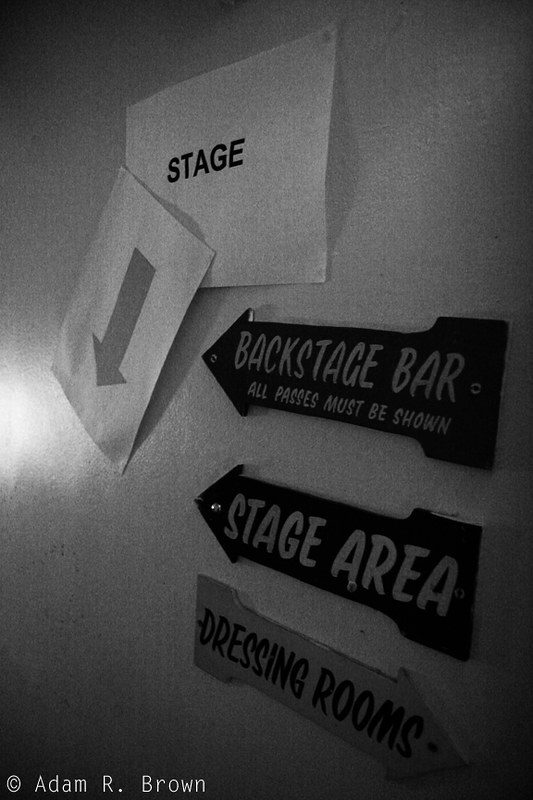In a dimly lit, monochromatic image dominated by shades of grey, white, and black, various signs are affixed to a wall located on the right side of a stairway, providing directions within a venue, possibly a concert hall. At the top of the image, a piece of paper with the word "STAGE" written on it hangs prominently, alongside an arrow pointing downward, indicative of a stairway below. Adjacent to this, on the left, another sign reads "BACKSTAGE BAR" with a left-pointing arrow, followed by an essential notice: "ALL PASSES MUST BE SHOWN." Below these, a directional sign labeled "STAGE AREA" also points left, while a final arrow labeled "DRESSING ROOMS" directs to the right. The bottom left corner of the image bears the name "ADAM R. BROWN" accompanied by a copyright symbol, indicating the creator of this photograph or artwork.